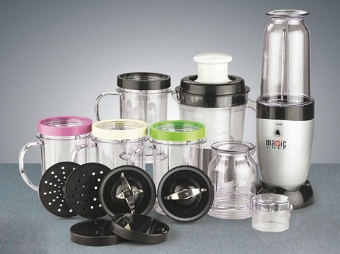The image is a detailed product photograph of a Magic Bullet Nutriblender displayed with an array of attachments and accessories. Central to the composition is the main blender unit, featuring a silver body with a black base and rim, subtly displaying the brand's logo on the front, though it is somewhat illegible due to the image's small size. Surrounding the main blender are multiple components: various blade attachments, personal cups with differently colored rims (pink, white, and green), and a measuring cup with different sizes for precise ingredient measurement. Also included are two additional types of blades and two types of strainers, both black and slotted, with matching solid covers. The entire setup is meticulously arranged on a gray granite countertop, against a plain gray background, suggesting it is prepared for a product advertisement. The clear glass cups and pitchers enhance the aesthetic appeal of the display. The image, seeming to serve as a thumbnail for a larger web depiction, encapsulates the versatility and accessorized completeness of the Nutriblender.